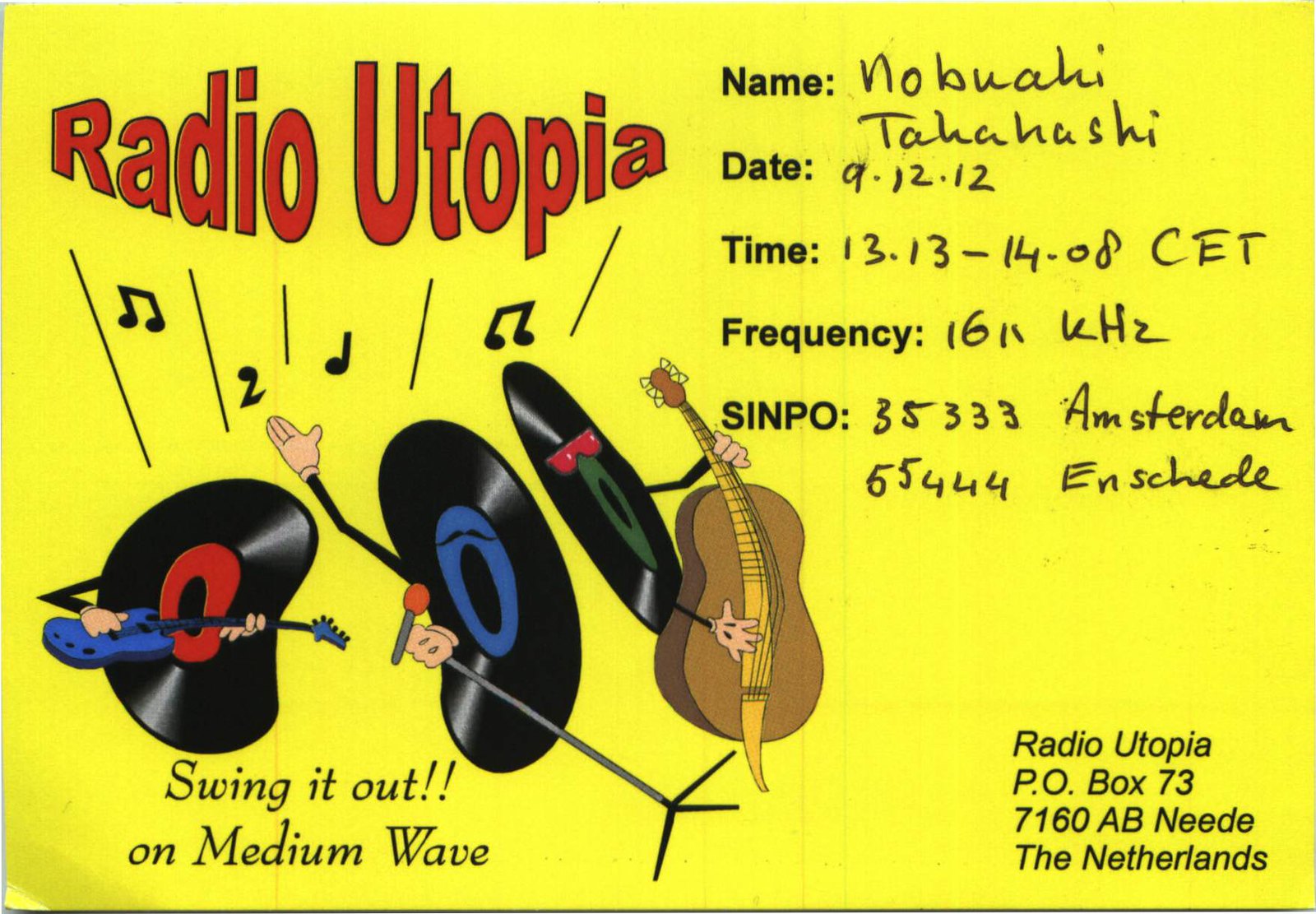The image is a horizontally aligned rectangular card with a solid yellow background, featuring subtle vertical gray lines in the middle, giving it a postcard-like appearance. In the upper left corner, large red letters spell out "Radio Utopia," beneath which are musical notes and a cartoon illustration of three records playing instruments: one record is playing an electric guitar, another is holding a microphone, and the third wears sunglasses and is playing a violin. 

Below the illustration, black text reads, "Swing It Out!! on medium wave." The upper right corner of the card contains fields for "Name," "Date," "Time," "Frequency," and "SINPO," all filled out in black ink: "Name: Nobuo Aki Takahashi," "Date: 9-12-12," "Time: 13:13-14:08 CET," "Frequency: 16 KHz," "SINPO: 35333," with additional annotations "Amsterdam 65444" and "Enschede." 

In the lower left corner, the image appears bent slightly, adding to its postcard feel. The lower right corner displays an address in black print: "Radio Utopia, P.O. Box 73, 7160 A.B. Neede, The Netherlands."